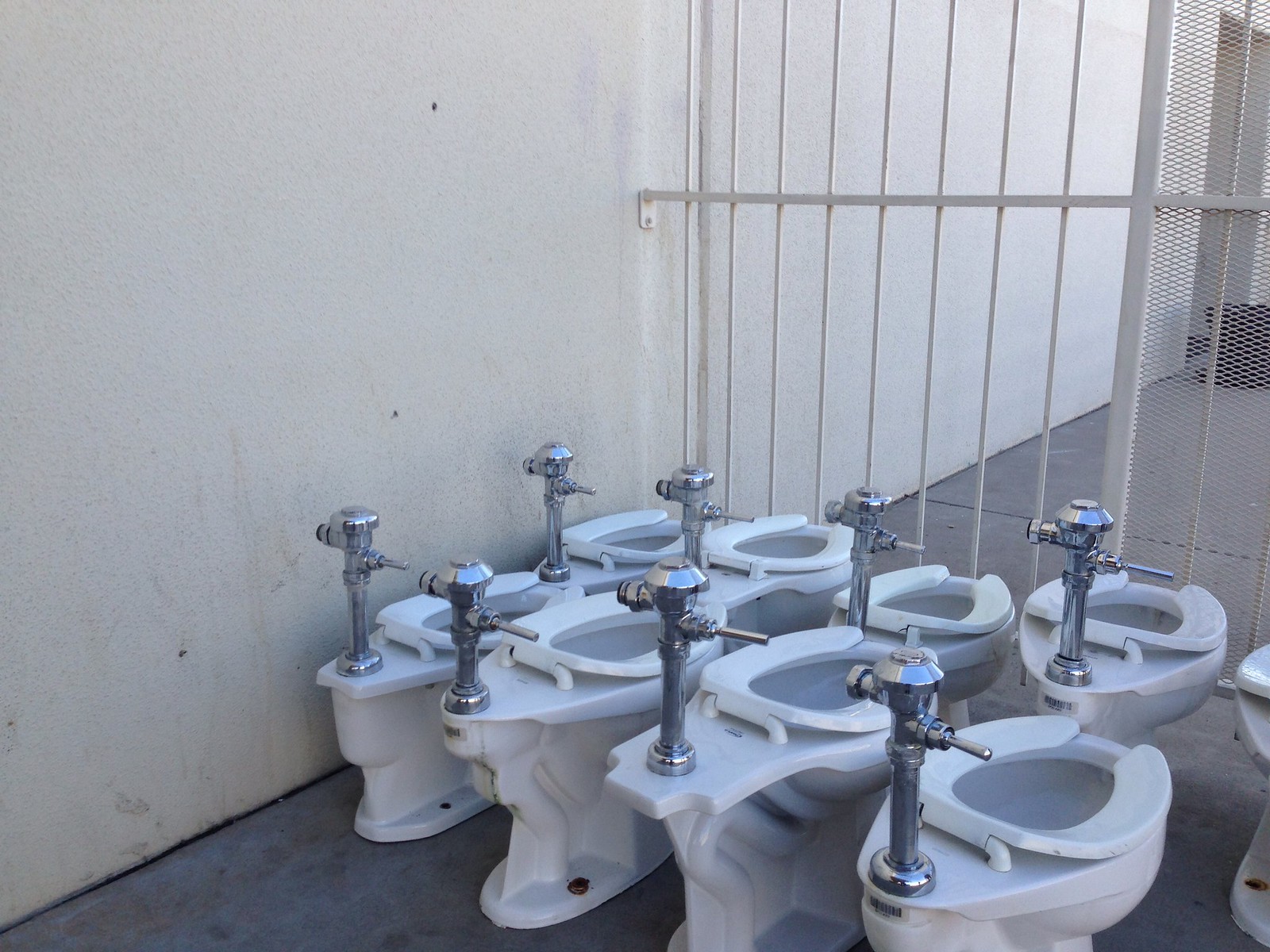The photo depicts an outdoor area that somewhat resembles a jail or prison yard, but it could also be another institutional setting. The scene features nine white porcelain toilets that are not connected to plumbing, all equipped with silver stainless steel pipes rising from the back. Eight of these toilets are clearly visible, arranged in two rows of four, with a ninth toilet partially visible at the edge of the photograph. The depicted area is divided by a metal fence with vertical bars and a grated section, creating a fenced-in area. The ground is covered in gray concrete, and the back of the area is defined by a stark white wall, which appears somewhat dirty and stained. In the upper right corner of the image, a door or doorway is visible, further emphasizing the institutional atmosphere of the setting. The toilets, lacking tanks, are reminiscent of those found in public restrooms, with flush mechanisms operated by stepping on the silver pipes.